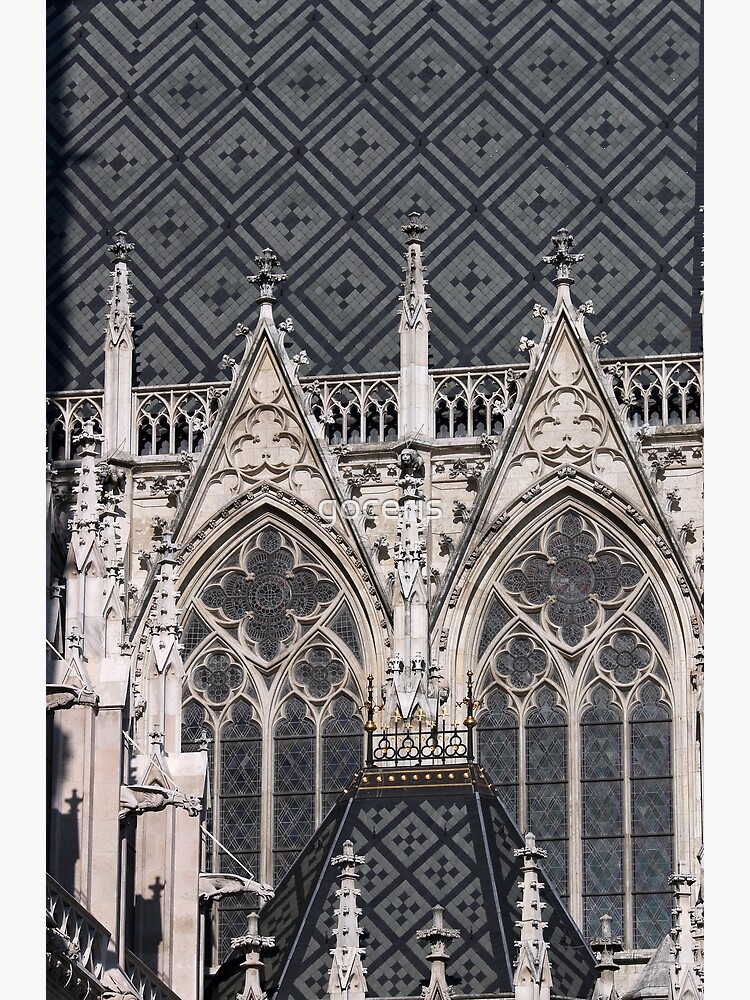The image depicts the ornate exterior facade of a church, highlighting its intricate architectural details and blend of colors. Prominently featured at the top are a series of checkered gray and black patterns resembling little boxes, situated above an elaborately decorated section that could be above the main entrance. This ornate section includes two pointy tips with black, beige, and brown filigree, complemented by steeple-like structures flanking the pointed areas. The facade also showcases detailed cathedral windows with stained glass featuring intricate floral designs. Each arched window culminates in a pointed top adorned with crosses and intricate patterns. The colors in the photograph are predominantly beige, brown, gray, black, and a touch of white. The roof is black, with elements of white wood framing parts of the structure, possibly including posts and fencing suggesting a balcony. The combined details of checkered patterns, filigrees, pointed structures, and decorative windows contribute to the overall ornate and pretty design of the church's exterior.